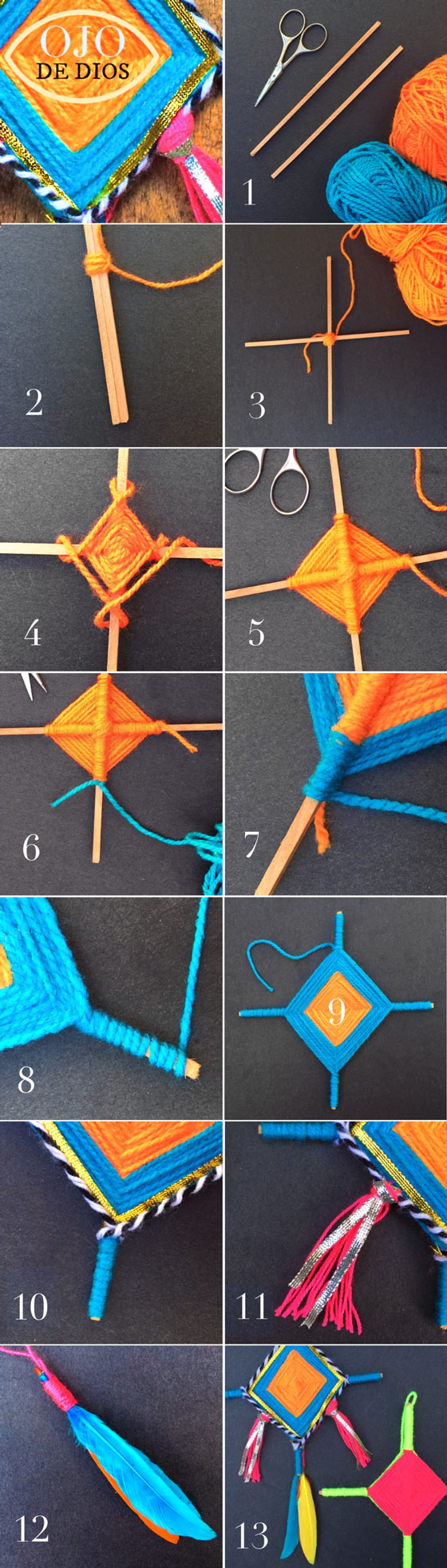This vertically oriented image, set against a black background, is divided into 14 square-shaped boxes, depicting a step-by-step guide for creating a yarn handcraft called "Ojo de Dios" (Eye of God in Spanish). The top-left box contains the title, while the remaining 13 boxes, numbered from 1 to 13 in white text, are arranged in 2 columns and 7 rows. The craft involves two sticks assembled in a cross shape, with orange and blue yarn threaded to form a diamond pattern at an angle. Detailed instructions visually guide the viewer through each step, showcasing the wrapping process of the yarn to create an intricate design with a center that resembles a kite or a Native American artistic piece. The final product includes tassels and feathers, with prominent orange and blue hues, and an additional red and green variation depicted in the bottom right box. Scissors and other art supplies are also mentioned within the instructions.